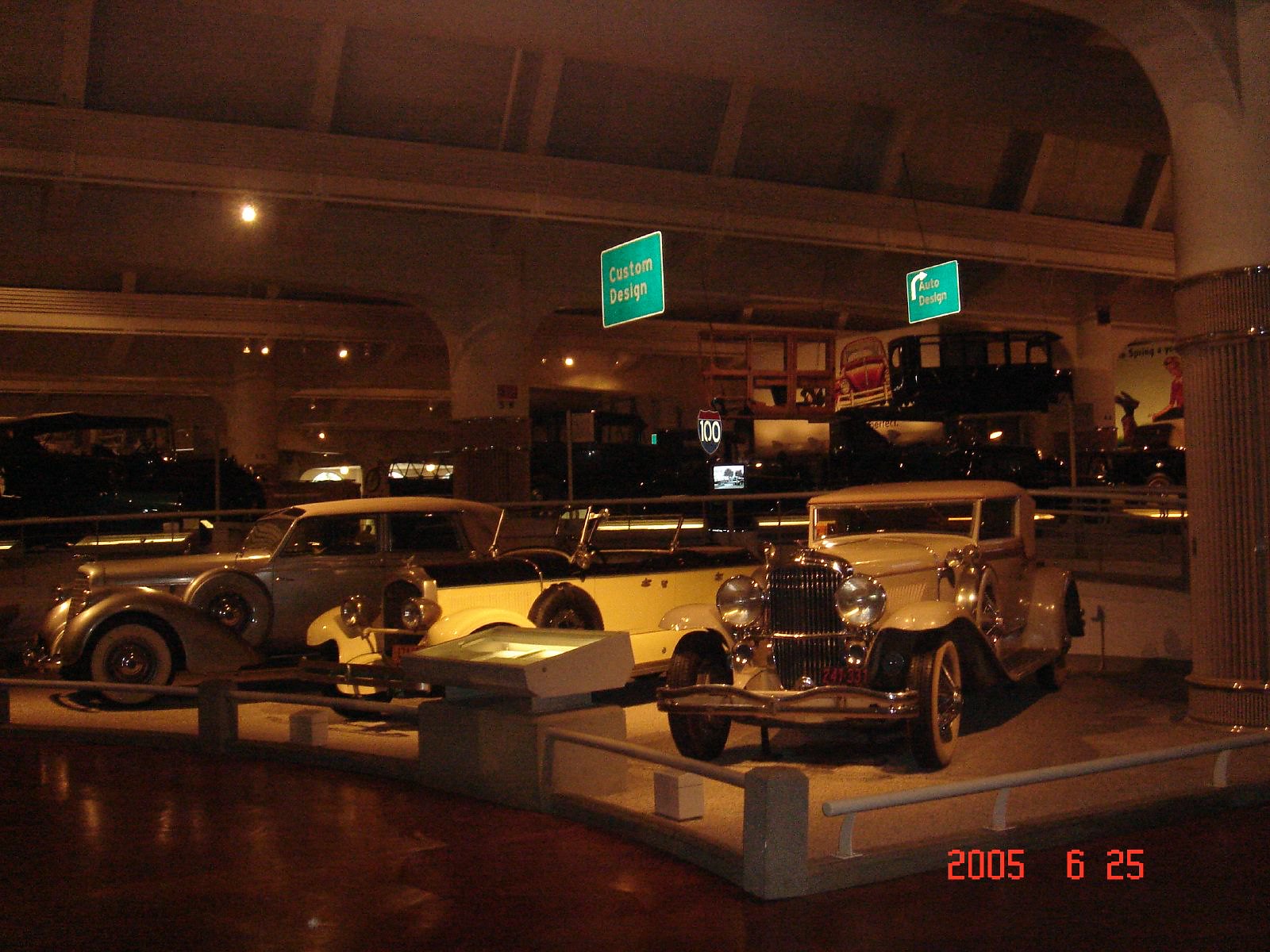The photograph showcases a dimly lit room, possibly within an automotive museum, filled with vintage luxury cars from the 1920s or 1930s. The setting casts a shadowy ambiance with subtle illumination from overhead lights, highlighting the reflections on the cars' bumpers and headlights. In the foreground, three prominently displayed vehicles in yellow and beige hues are positioned at angles—one to the left, one diagonal, and one toward the center—each situated within their own partitioned showroom space. Overhead, green and white street-sign-shaped indicators hang, one reading "Custom Design" with an arrow pointing into the room. The display area features a cement-colored stone floor and no visible people, emphasizing the cars as the central focus. Additionally, a dated timestamp "2005-625" is visible in the bottom right corner of the image, adding a historical context to the scene.